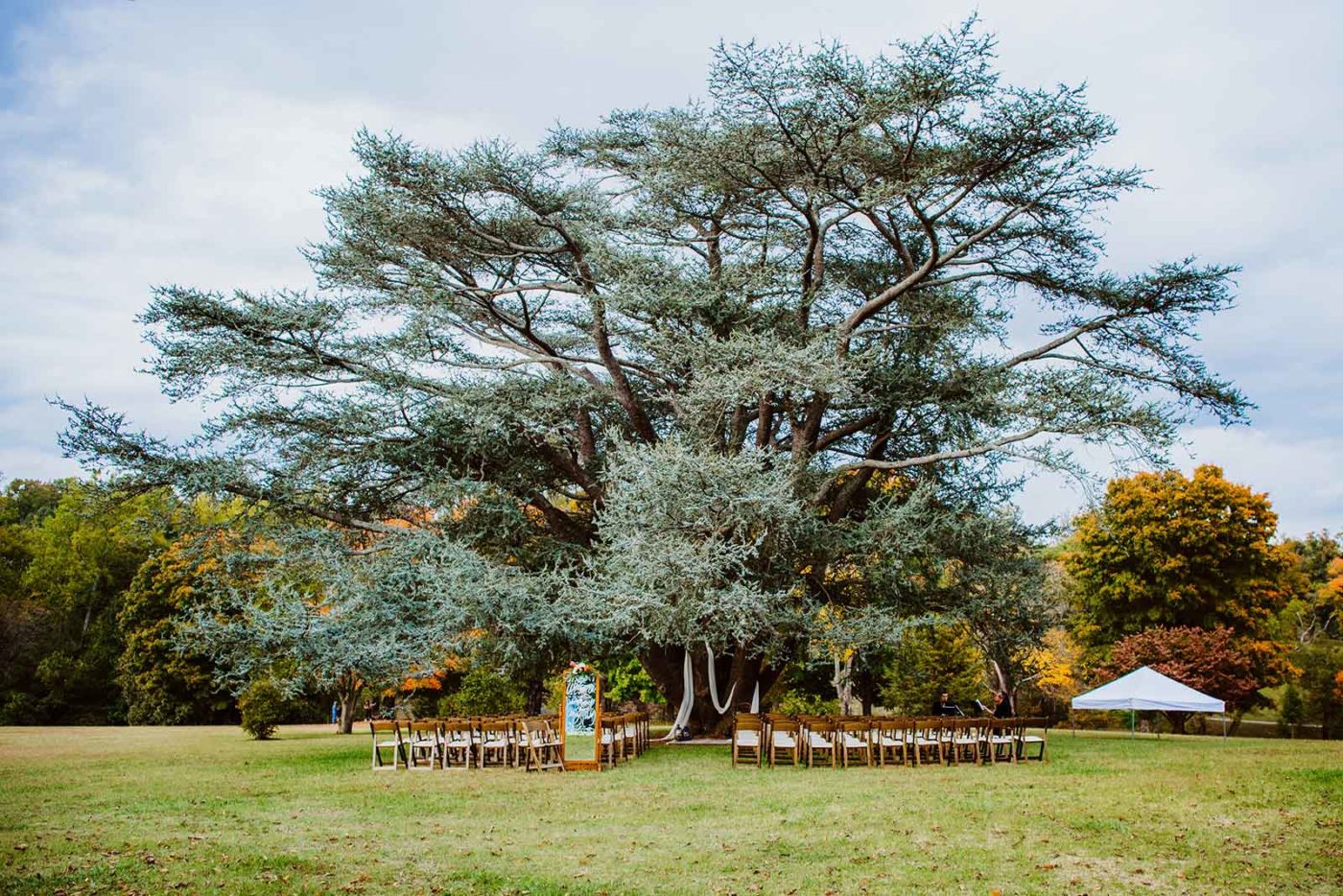The image captures a beautifully serene scene in what appears to be a park, meticulously arranged for an outdoor event, likely a wedding. In the center of the frame, a majestic, sprawling tree with enormous branches, possibly an old oak, commands attention. The tree's verdant leaves stand in contrast to the autumn-hued foliage of the surrounding trees, with colors ranging from green to yellow, red, and brown, suggesting a seasonal transition. Beneath the tree, rows of wooden chairs with white seats are neatly arranged on lush green grass, forming two lines with a central aisle, leading towards what might be a platform for the ceremony. To the right, a white canopy tent is set up, hinting at additional preparations for the event. A white cloth draped from one of the tree's branches adds a touch of elegance to the already picturesque setting. The sky above is partly cloudy and hazy, casting a soft light over the scene, void of strong shadows, enhancing the tranquil ambiance. The overall setup exudes a sense of anticipation and beauty, perfect for a special celebration amidst nature.